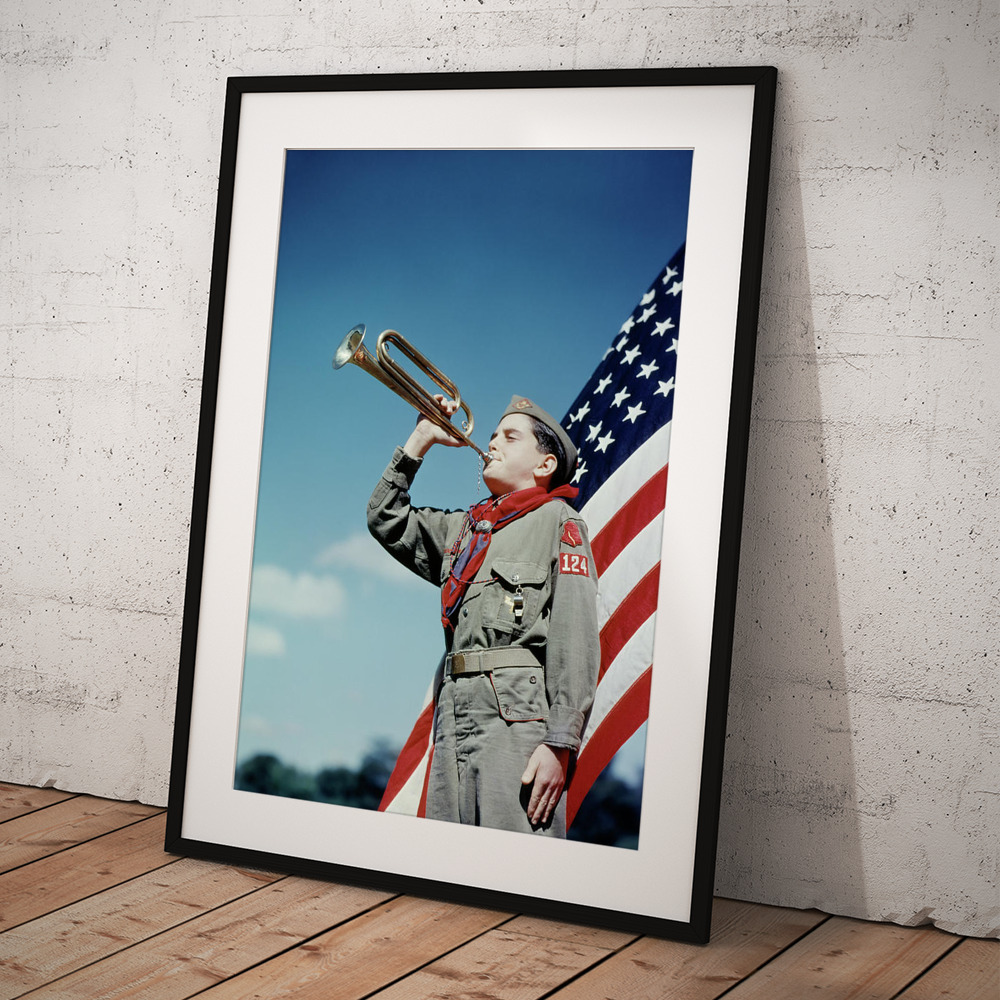A framed photograph rests on a wooden plank surface, leaning against a plastered wall that appears to be covering brick. The frame is simple and black, with a white mat that emphasizes the patriotic scene within. The photograph captures a young Boy Scout, likely around 10 or 12 years old, standing at attention. He is dressed in a pale green khaki uniform adorned with a red scarf and a badge on his left sleeve displaying the number "124". His right hand is raised as he blows into a bugle, and his left hand hangs straight down by his side. The Boy Scout wears a matching pale green hat and stands proudly before a waving American flag, which can be seen in the background along with elements of a blue sky and blurred trees. This evocative image, brimming with patriotism, is beautifully framed and propped against the textured wall, creating a striking display.